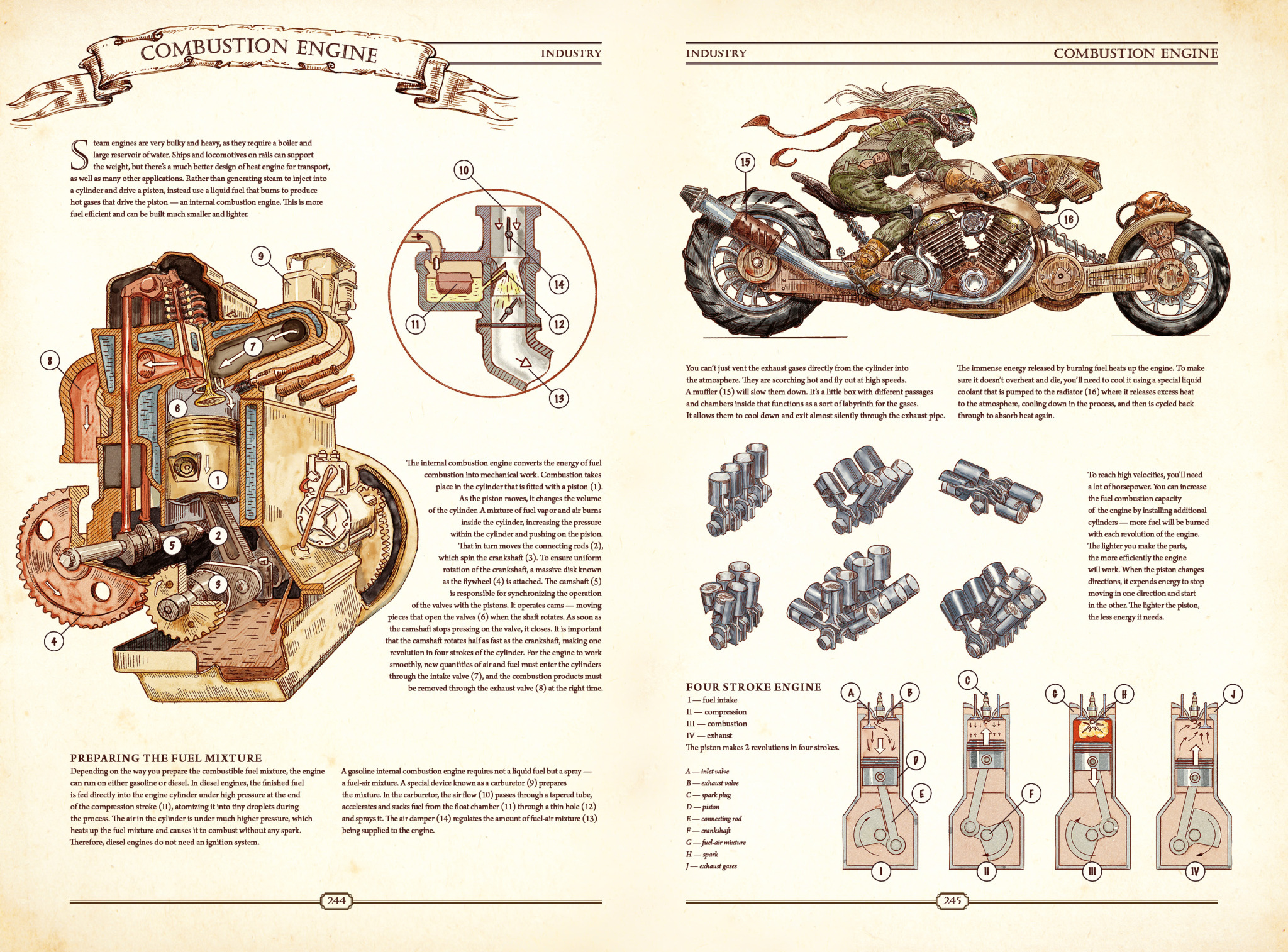The image depicts a colorful two-page spread from a vintage book or magazine, focusing on the design and mechanics of combustion engines. On the left page, a banner at the top reads "Combustion Engine" with the word "Industry" flanked by vertical rules. Below this, a detailed paragraph explains the efficiency and compact nature of internal combustion engines compared to steam engines. A large, intricate color illustration dominates the page, showing a beige, rust, and blue engine with its interior parts labeled and referenced by numbered blowout circles. A smaller, magnified view of a segment of the engine appears in a brown-outlined circle, similarly numbered. The bottom of this page includes instructional text and diagrams, outlining the four-stroke engine process: intake, compression, combustion, and exhaust, along with labeled engine components like the inlet valve, exhaust valve, and spark plug.

The right page features a vivid profile view of a fantasy illustration with a dragon-faced creature, adorned in camo attire and a flowing scarf, riding an extended motorcycle. The motorcycle, with its rust and bronze engine and visible silver metallic pistons, contrasts against the creature's green outfit and red neck ribbon. The text once again labels the "Combustion Engine" and "Industry," with precise diagrams of engine valves and parts labeled with letters A through F, providing further detailed mechanical insights. Overall, the image combines educational technical drawings with imaginative art, creating an engaging, informative spread.